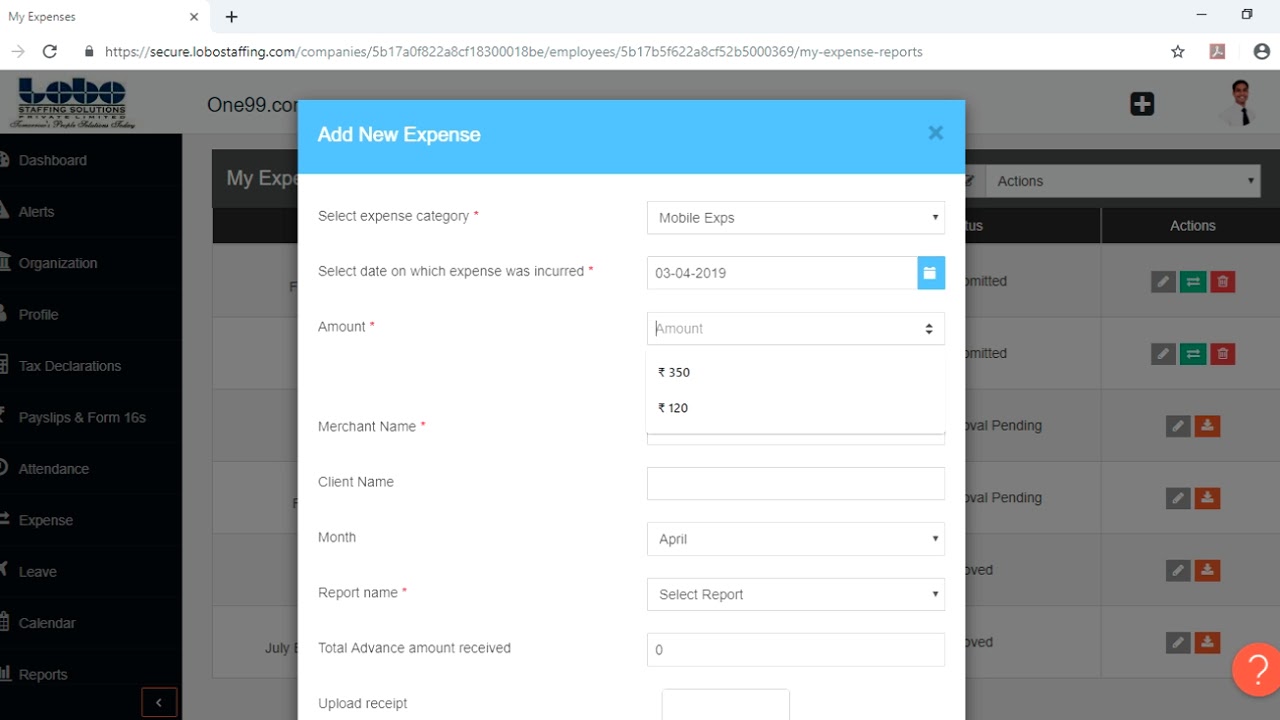The image depicts a web browser open to a secure webpage, specifically secure.lobostaffing.com, which belongs to Lobo Staffing Solutions. The browser tab is labeled "My Expenses." On the upper left-hand side of the webpage, the logo and name "Lobo Staffing Solutions" are clearly visible. To the immediate right, it also displays "199.com."

A vertical menu is situated on the right-hand side of the webpage, featuring various sections such as Dashboard, Alerts, Organization, Profile, Tax, Declarations, Pay Slips and Forms, Attendance, Expenses, Leave, Calendar, and Reports.

In the foreground, there is an active pop-up window titled "Add New Expense." This window includes multiple input fields: Select Expense Category, Amount, Select Date on which expense was incurred, and Merchant Name.